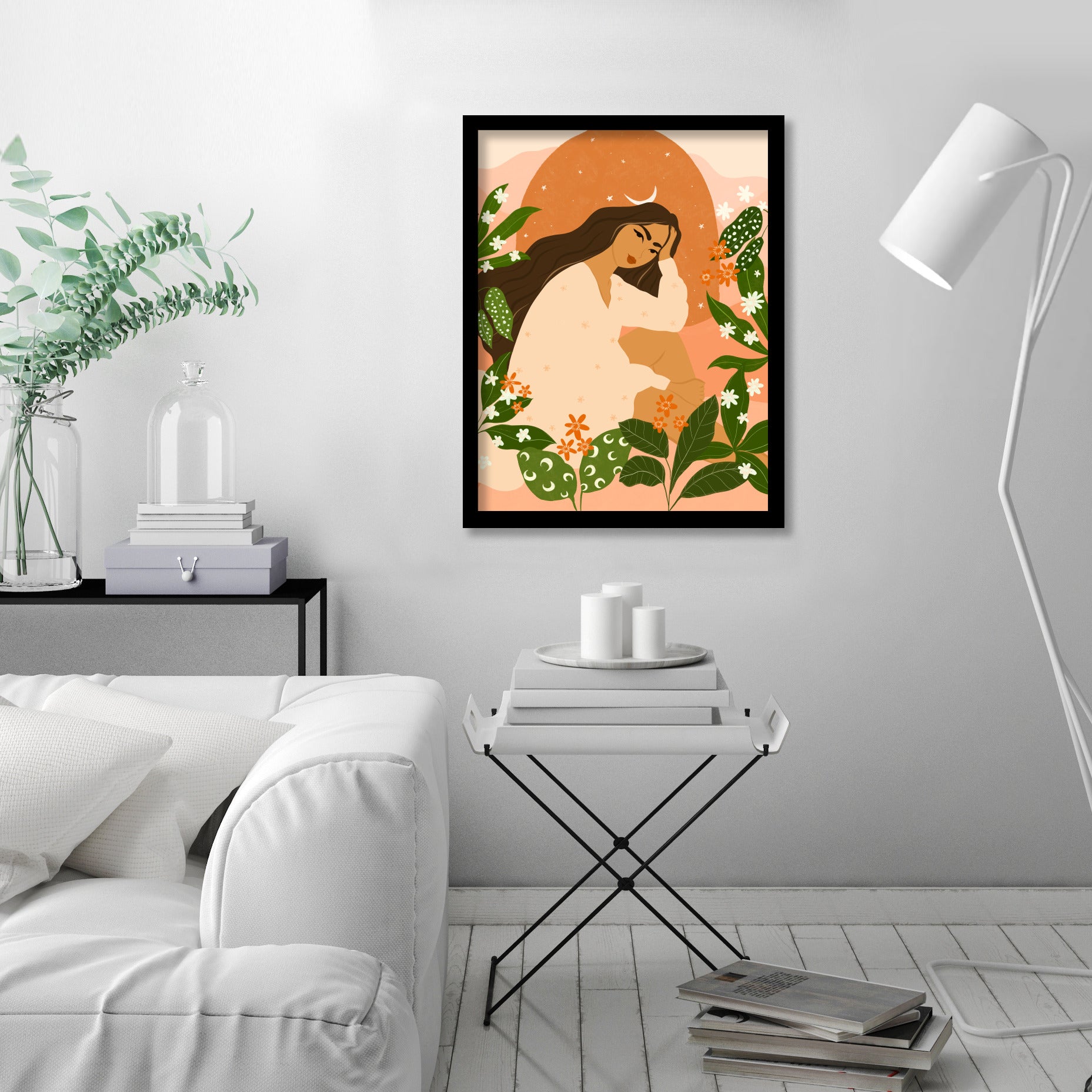The image captures a meticulously curated room with a predominant white and black color scheme. The walls and floor are stark white, providing a clean, minimalist backdrop. Centered on the wall is an evocative painting encased in a black frame. This painting features a woman with long, wavy brown hair, surrounded by green leaves speckled with white stars, and a crescent moon hanging over her head. The woman is depicted in a light coral dress, seemingly seated with one hand on her head.

To the left of the image, there's a white sofa adorned with two white pillows. Adjacent to the sofa on the right side is a tall, white lamp. A small table with a white top and crisscrossed black legs is positioned at the bottom center of the image, holding white books and what appears to be a white plate with a white candle. Additional books, in white and black, are scattered near the table on the floor.

On the right side, above the sofa, there's a black table pushed against the wall, displaying glass vases, one of which contains green plants. This refined arrangement of furniture and decorative elements creates a harmonious and visually appealing space.